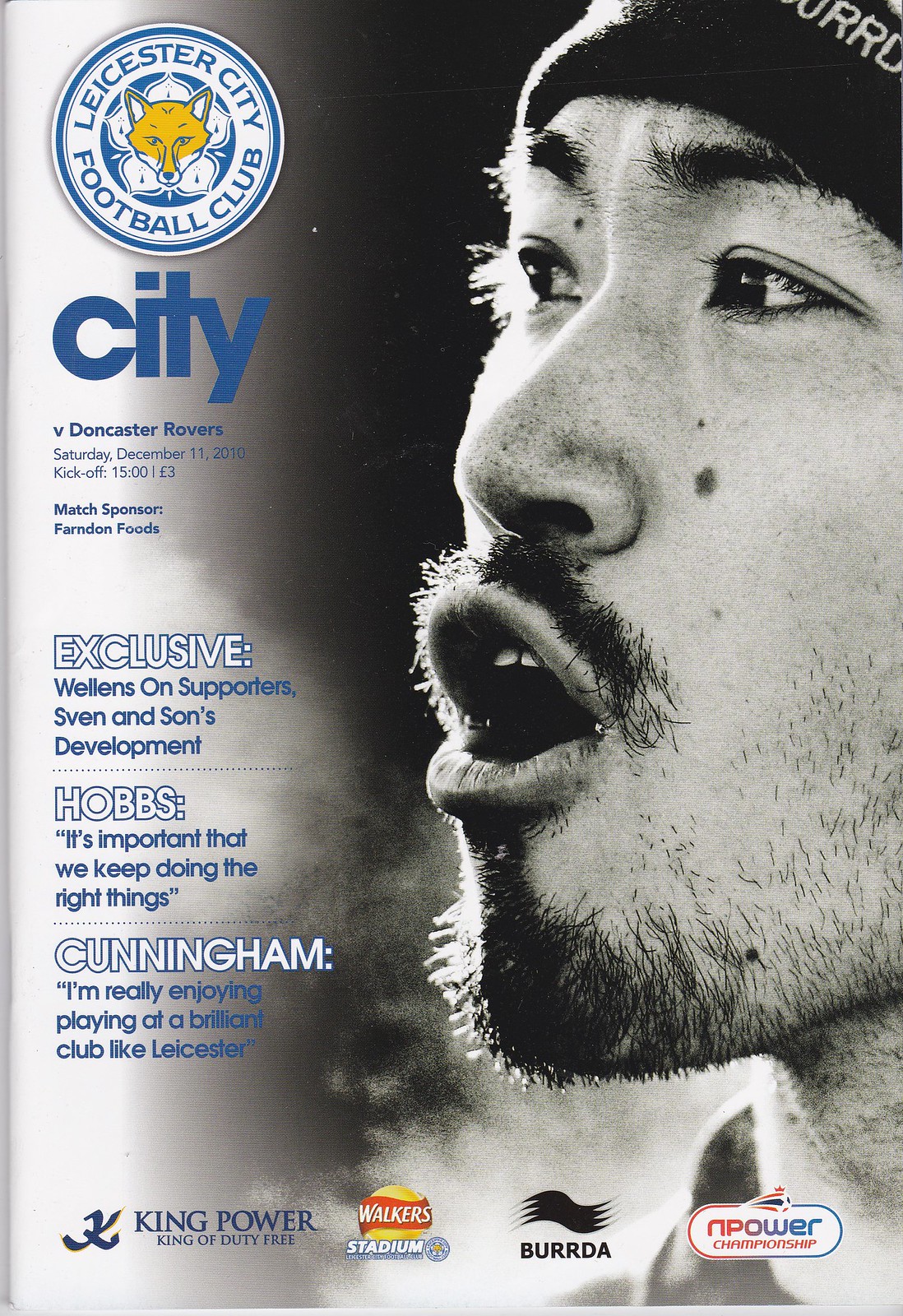The image appears to be the cover of a magazine, prominently featuring a close-up, black-and-white photograph of an Asian man’s face, extending from slightly past his eye to the right-hand side of the cover. He sports a short black mustache, a goatee, and stubble, with dark eyes and black eyebrows, and is wearing a black hat. His mouth is open, possibly in mid-speech or shout.

In the upper left corner, there is a circular logo with a blue outline and a yellow fox in the center. It reads "Leicester City Football Club" and below the logo, "City" is written in bold, blue letters. Beneath this, in smaller blue print, the text details, "V Doncaster Rovers, Saturday, December 11, 2010, kick-off: 15:00, L3." Further down, it notes "Match Sponsor: Fern Dun Foods."

On the left side of the cover, in large white letters outlined in blue, is the word "EXCLUSIVE." Below this, in blue text, it states, "Wellens on supporters, friends, and Sons' development..." with a line of dots trailing off. Directly beneath, in white text outlined in blue, it reads "HOBBS," followed by a quote in blue: "It's important that we keep doing the things..." and another line of dots. The name "Cunningham" appears below the quote, followed by smaller blue text stating, "I'm really enjoying playing at a brilliant club like Leicester."

At the bottom of the cover, underneath the athlete's chin, there are several logos of sponsors, including King Power, Walkers, Beretta, and N-Power.